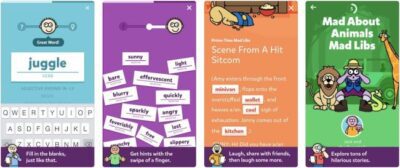Sure! Here is the cleaned-up and detailed descriptive caption:

The image displays a series of four screens arranged horizontally. 

1. **First Screen (Left)**: The background is light blue with a prominent white rectangle in the center featuring the word "JUGGLE" in capital letters. There is an emoji face present, though the text it displays is illegible. A virtual keyboard is overlaid on the bottom part of the screen. There is also a purple element and another cartoon character next to the keyboard, but their messages are not clear due to poor resolution.

2. **Second Screen**: This screen has a purple background and is filled with multiple overlapping white rectangles that contain text, though the exact words are unclear. One might contain "Quickly," and another, "Effers," but the text is not legible. The same emoji face from the first screen is present at the top, on a structure that resembles a slide, with parts in purple and others in white. Another character is visible at the bottom of the screen, depicted on a purple background, but its text is also unreadable.

3. **Third Screen**: The background color is light purple. The white rectangles and emoji face continue to appear, along with a structure that resembles a slide, which again includes both white and purple elements. The text in these rectangles remains unreadable.

4. **Fourth Screen (Right)**: The background is orange and prominently features the text "Scene from a Hit Sitcom." Additional text is present but is illegible.

Overall, the poor resolution of the images makes it difficult to accurately ascertain the exact text and details presented by the emoji faces and characters.